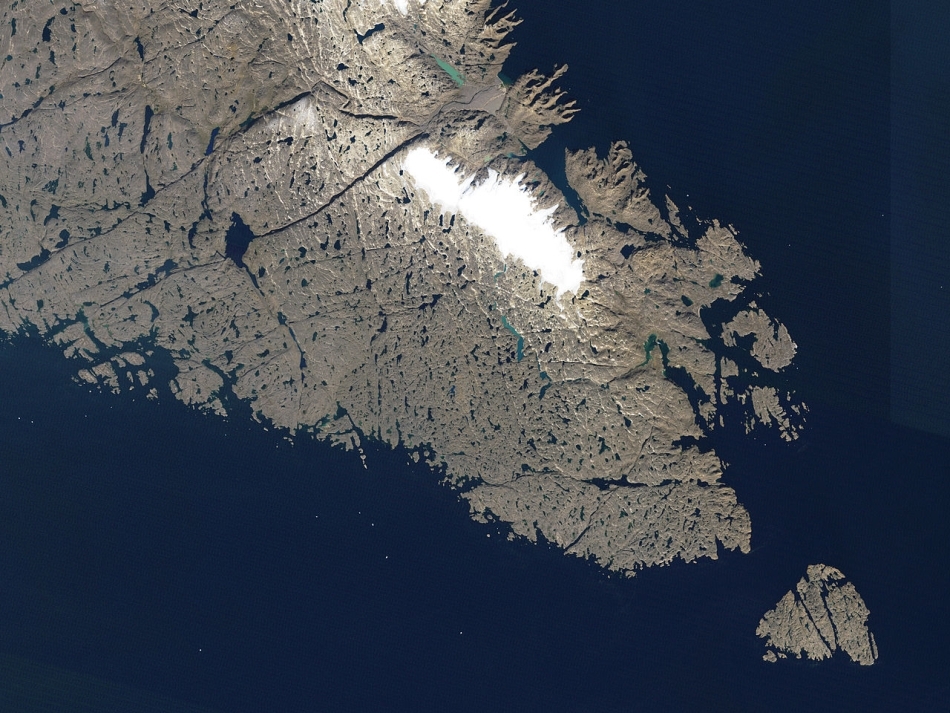This is a detailed color aerial photograph, likely a satellite image, capturing a long, beige peninsula extending from the upper left-hand corner toward the lower right-hand corner of the rectangular frame. The peninsula's elongated form resembles a pointed tail cutting across the image, surrounded by dark navy to black waters. Within the peninsula, numerous small bodies of water and potential canals and rivers are present. The upper right portion of the peninsula features a bright white area, suggesting either snow-capped peaks or a reflective surface. Beyond the peninsula, near the bottom right corner, an isolated triangular island emerges from the water, further emphasizing the complex interplay of land and sea in this striking geographic landscape. The overall scene evokes the image of a colossal tail adorned with white spikes, reminiscent of Godzilla's iconic form.